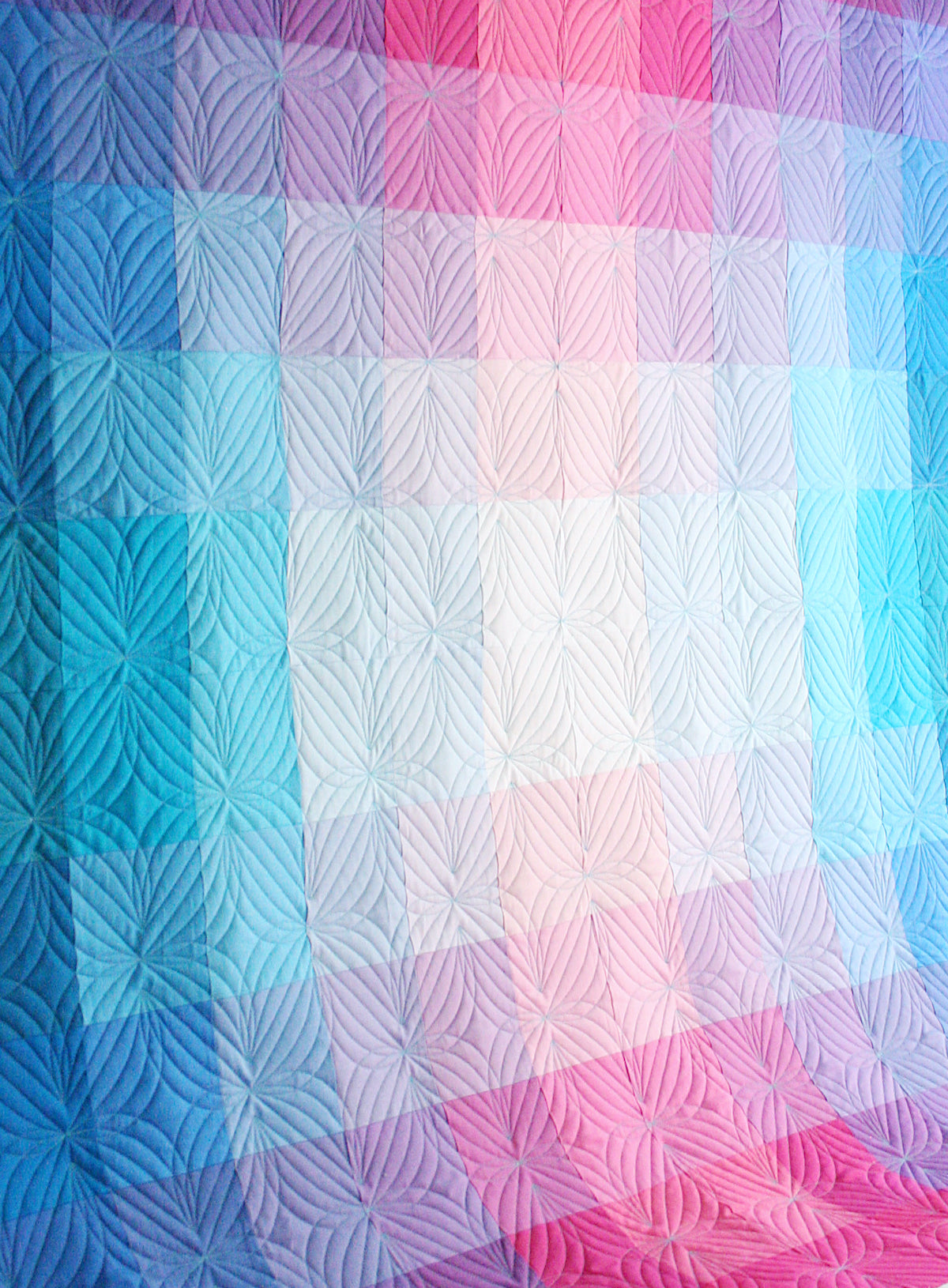The image showcases a vertically oriented, vibrant patchwork quilt resembling a four-petaled flower. The intricate design features numerous square-shaped patches arranged in a colorful gradient. Starting from the leftmost column, the quilt displays dark blue squares transitioning to lighter blue hues towards the center. Moving rightward, the colors shift progressively through various shades of purple, pink, and red, culminating in the central columns which consist of lighter shades including light blue, turquoise, light pink, and white. The top and bottom sections mirror these transitions, with purples and pinks blending into the brighter, central white patches. The quilt radiates a bright and vibrant palette, illuminated by natural light, making each color and detail vividly clear.